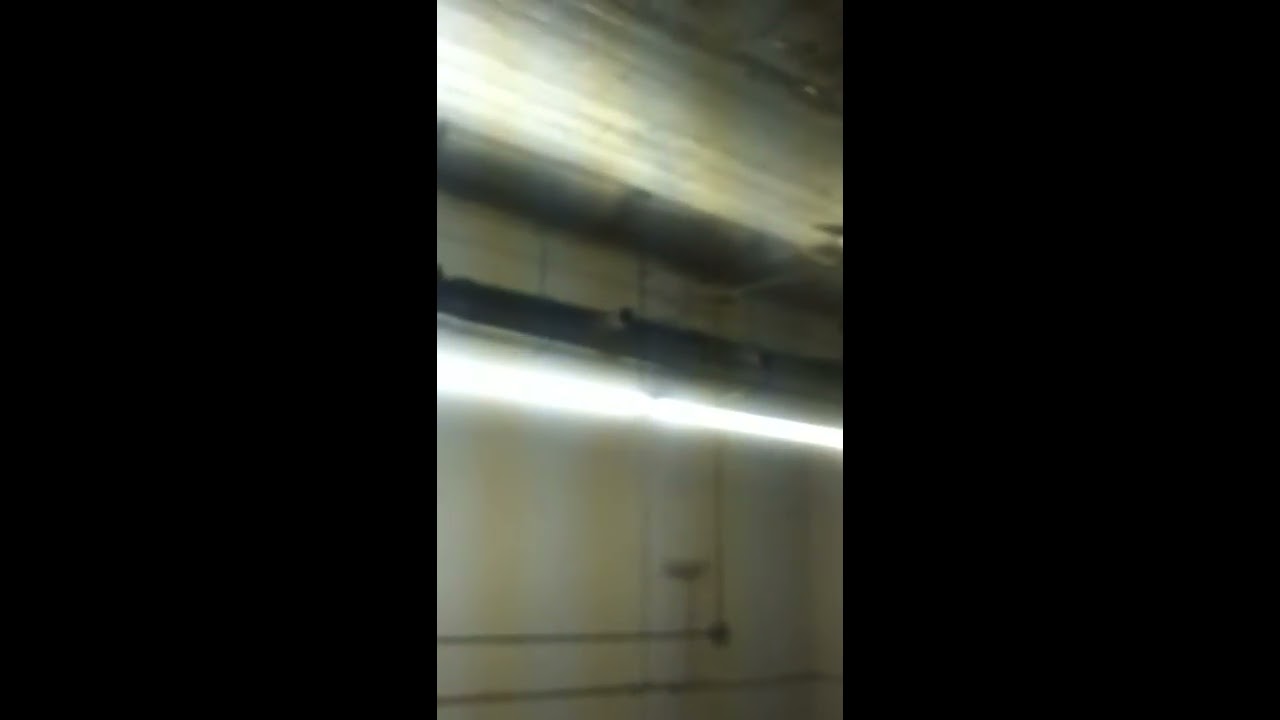The image presents a detailed and somewhat gritty view of the interior of an industrial or commercial space, possibly a factory or warehouse. The main focal point is the white wall, which is prominently stained with vertical yellowish lines, indicating age and possible water damage. There's visible electrical conduit piping running horizontally across the wall. The ceiling, sharing a similar white hue with the wall, also displays these yellow streaks, adding to the overall aged appearance of the space. Several fluorescent tube lights are mounted horizontally on the wall, casting a brighter glow on the left side of the image. Near the top of the ceiling, there is ductwork or a ventilation system with a mixed black and white color scheme. Overall, the photograph, despite its blurriness, conveys a sense of industrial wear and utility, emphasizing the stark and functional design elements like the hanging lights and exposed pipes.